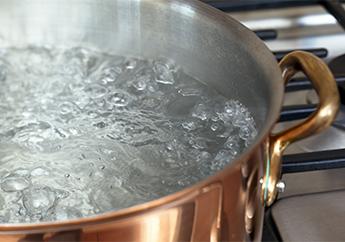The image depicts a close-up view of a copper pot, characterized by its bronze exterior and silverish stainless steel lining, situated on a gas stove. The pot is filled with clear water that is rapidly boiling, indicating that the stove has been on for some time. The right side of the pot features a copper or metal handle adorned with several rivets. Surrounding the pot, a part of the black metal grate of the stove is visible, and in the background, the rest of the stove, possibly made of stainless steel, can be seen. There is a noticeable highlight on the pot and inside it, suggesting the use of a flash during the photo capture.